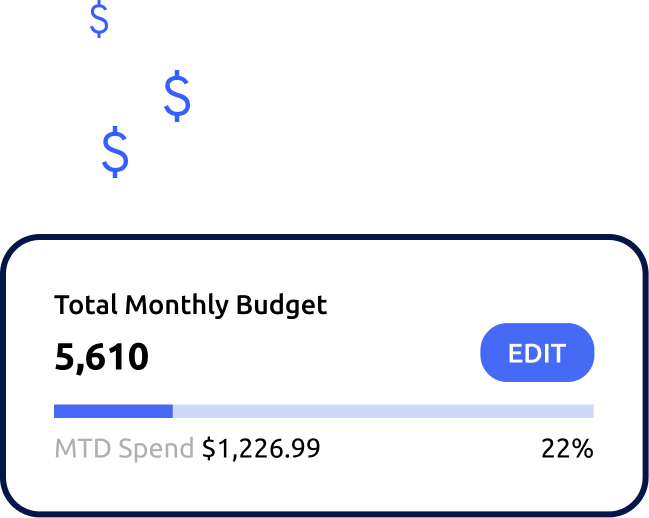The image is a screenshot taken from a website, which displays a monthly budget breakdown. The screenshot is cropped just below the address information section. At the top of the image, there are three blue dollar signs arranged in a staggered, vertical fashion. The dollar signs are not highly detailed; two of them are similar in size, while the third is noticeably smaller.

Below the dollar signs, there is a large rectangle with rounded corners, outlined in a dark black line. Inside the rectangle, "Total Monthly Budget" is written in bold black font. Directly below this text, the total budget amount of $5,610 is displayed. To the right-hand side of the rectangle is a blue button with white text that reads "Edit."

Underneath this section, the first line item of the budget is listed, showing an expenditure of $1,226.99, which accounts for 22% of the total budget.